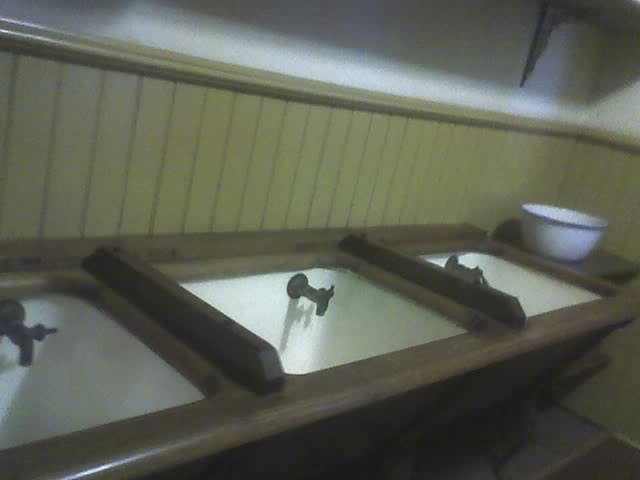The image captures a slightly blurry interior shot at an angle, focusing on a trio of white sinks with black faucets, each attached to a wooden countertop. Positioned to the right of these sinks is a white bowl with black trim, resting on a small wooden stand. Behind the sinks, a wooden-paneled wall with vertical stripes serves as a backsplash, contrasting with the off-white upper portion of the wall where a shelf bracket casts a shadow. The wooden countertop features divisions between the sinks, aligning with the blend of rustic and minimalist design elements in the space. The overall setting is warm and cohesive, with the greenish paneling and wooden textures adding depth to the decor.